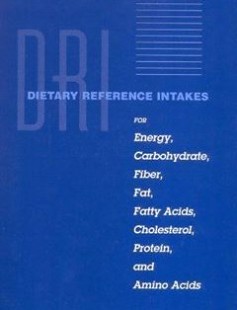The cover of the book, likely a brochure or medical reference guide, features a medium-dark blue background with no images. Prominently, it displays the acronym "DRI" in large, opaque letters. Above this, in light blue text, it reads "Dietary Reference Intakes." On the top left corner, there's a simple geometric pattern composed of horizontal light blue stripes arranged in a square shape. Below "Dietary Reference Intakes," in white text, the book lists: "for energy, carbohydrate, fiber, fat, fatty acids, cholesterol, protein, and amino acids." The minimalist design underscores its professional and educational intent.